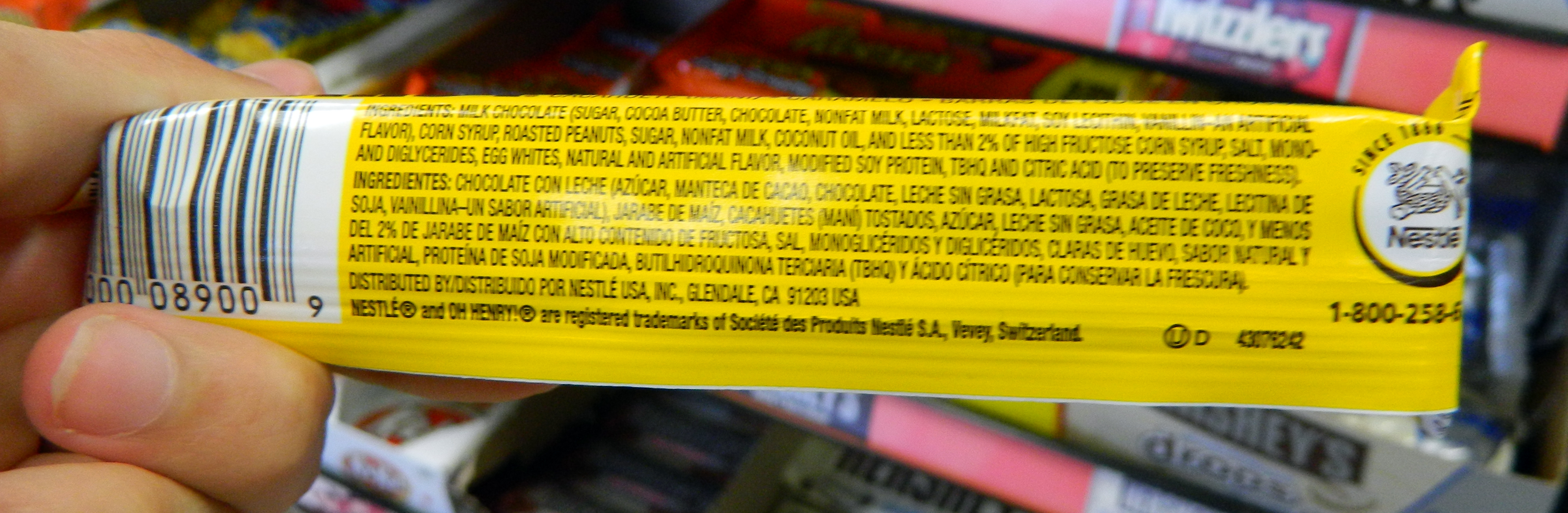This close-up photograph captures a Caucasian man's hand holding a yellow-labeled Nestlé O'Henry candy bar, showcasing its back side. Prominently featured are black-printed ingredients listed in both English and Spanish, including milk, chocolate, sugar, cocoa butter, and other more specific components. The label also exhibits a black-and-white barcode on the left and a distinctive white Nestlé logo encircled on the right, accompanied by a 1-800 phone number for the company. Fine print at the bottom identifies Nestlé O'Henry as registered trademarks of Societe de Product Nestlé Vervis, Switzerland. In the background, the vibrant scene includes an array of other candy items like Twizzlers, Hershey's, Kit Kat, Reese's Cups, and a distant Butterfinger, suggesting the setting is a store's candy display near the checkout area. The man's fingers are visible holding the candy bar's left end, indicating an engaged and tactile inspection of the item's packaging.